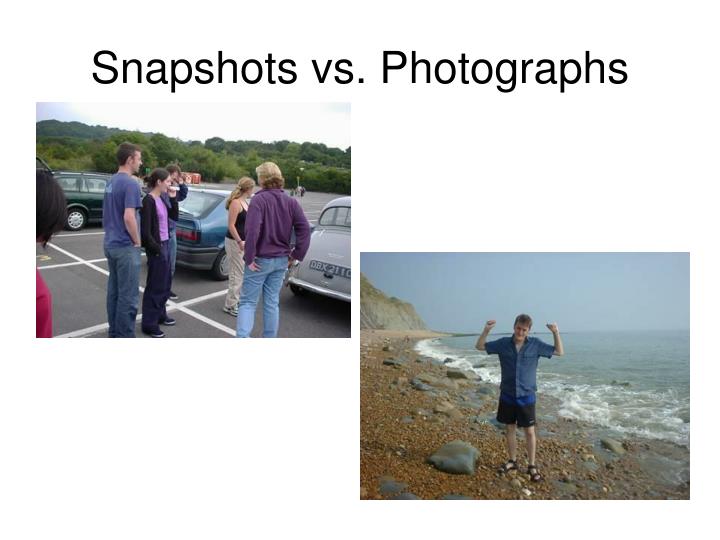This image appears to be a slide from a presentation comparing snapshots versus photographs, as indicated by the black text at the top. The slide contains two photos arranged diagonally. 

On the left side, there is a candid snapshot of five individuals standing in a parking lot. They seem engaged in a conversation and are looking away from the camera, suggesting a casual, unposed moment. The setting includes several parked cars, trees in the distance, and a mixture of grassy and vegetative backgrounds, possibly indicating a location in Europe based on visible license plates. The group is dressed casually in varied attire, such as blue jeans, khakis, a purple hoodie, a black tank top, a purple top, and an indigo t-shirt.

On the right side, positioned somewhat lower, is a more intentional photograph of a single person standing on a gravel beach near an ocean. This individual is facing the camera and striking a triumphant pose with both arms raised, emphasizing a posed and purposeful photo. The young man, likely in his late teens or early 20s, is dressed in a blue button-down shirt, black shorts, and sandals. The backdrop features a cliffside to the left and a gray sky, contrasting with the whiter sky seen in the snapshot.

The contrast between the spontaneous casual group scene and the posed, celebratory solo shot illustrates the difference between snapshots and photographs, highlighting intent, composition, and engagement with the camera.